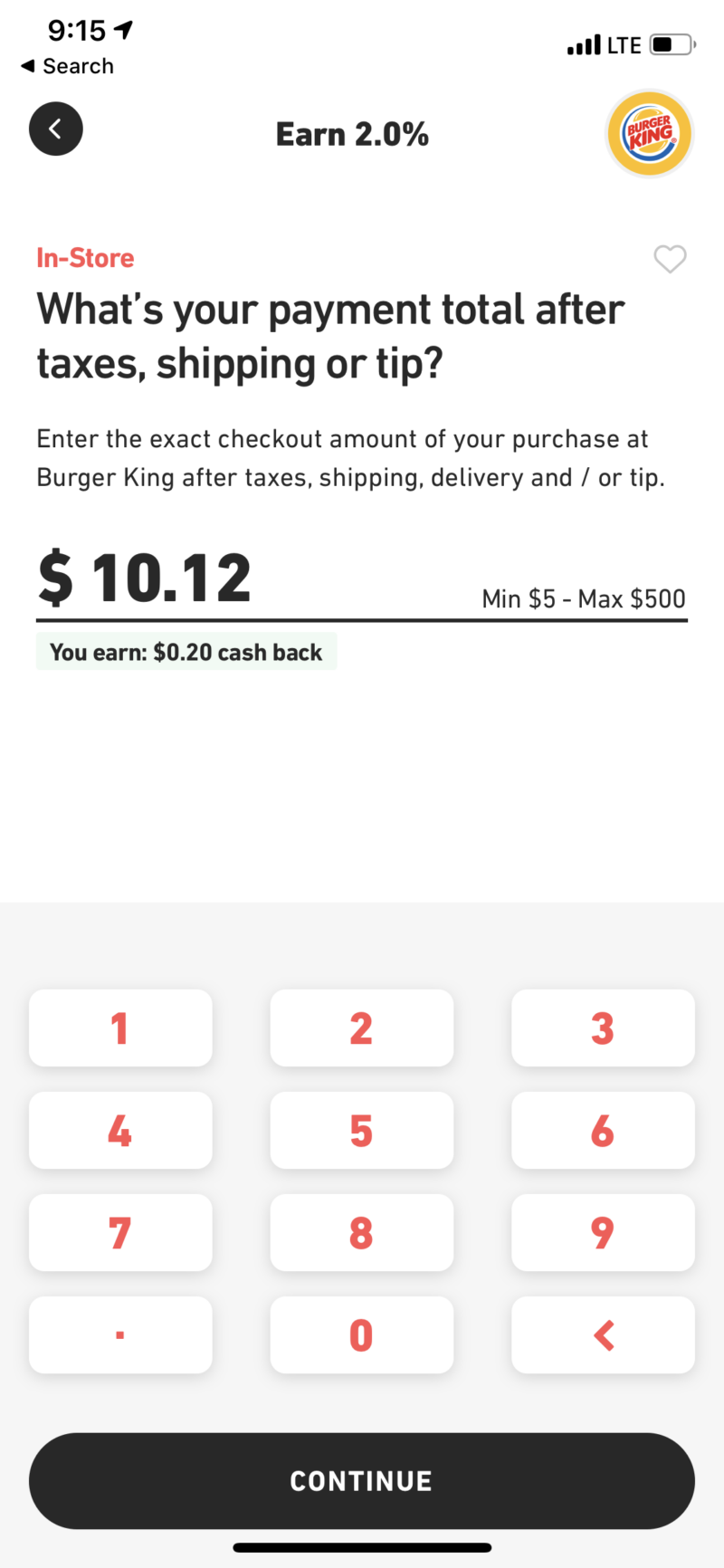The screenshot displays the interface of a mobile device at 9:15 AM, as indicated by the time in the top left corner. In the top right corner, the screen shows a fully connected network with 4 out of 4 signal bars, an LTE icon, and a battery level indicator.

The central section of the screen is occupied by a search application. At the top left of this section, there is text that partially reads "N2%". Below this, a prominent button labeled "Install" is visible.

Further down, the screen presents instructions for entering a payment amount. The text reads: "What's your payment total after taxes, shipping, or tip? Enter the exact checkout amount of your purchase at Burger King after taxes, shipping, delivery, and/or tip. $10.12. Minimum $5 to maximum $500."

At the bottom of this section, it notes that by entering the purchase amount, you will earn $0.20 in cash back.